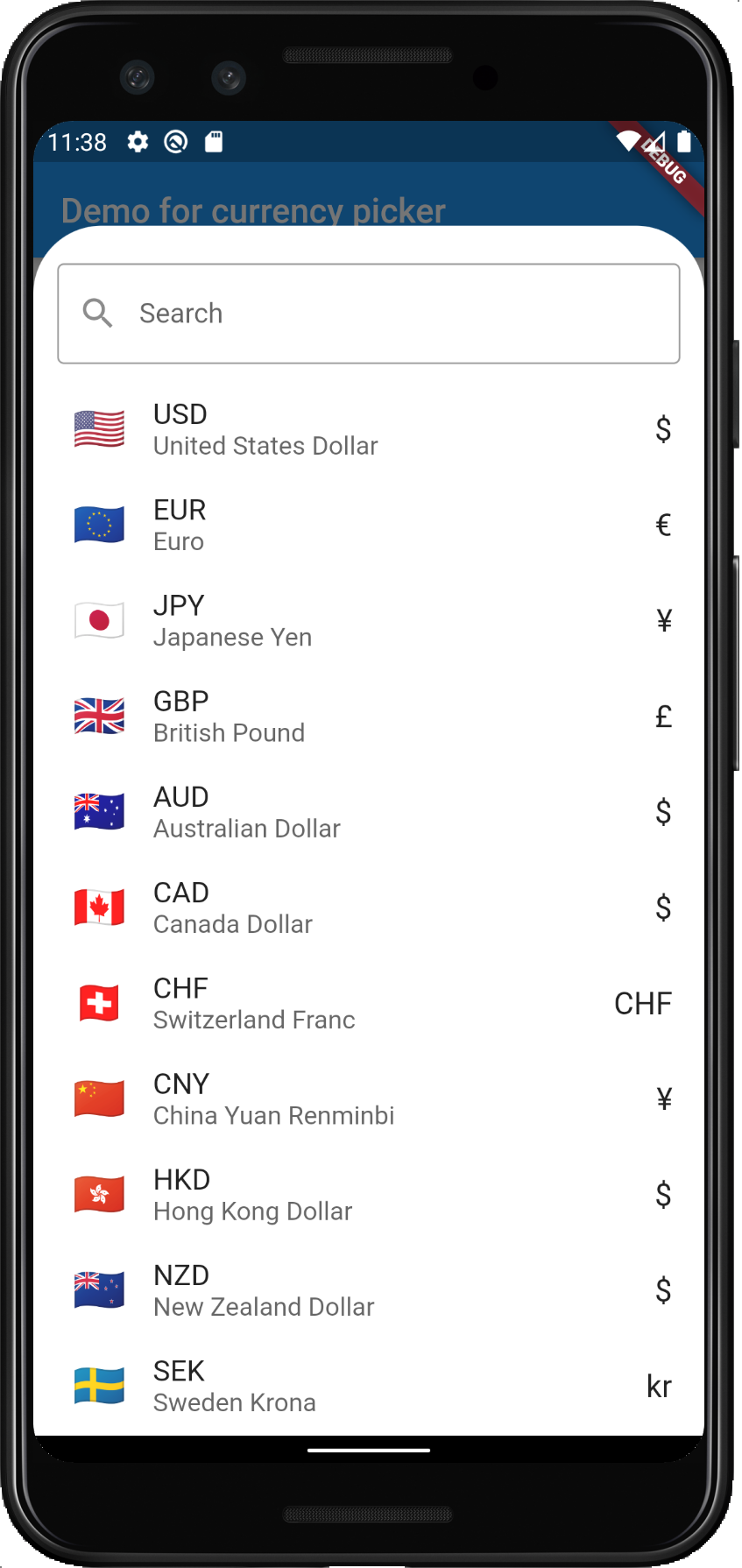The image displays a photograph of an iPhone, capturing its entire form rather than a simple illustration. At the top of the screen, the time is displayed as 11:38 against a blue-shaded section. In the upper right corner, there is a small banner with white lettering that is partly obscured by other elements. Below this banner, the text "Demo for Currency Picker" is prominently shown atop the blue section of the screen.

Central to the image is a white search bar situated beneath the blue banner. Below the search bar is a list of various countries and their corresponding currencies. The listed currencies include:
- U.S. Dollar (USD) with the symbol $
- Euro (EUR) 
- Japanese Yen (JPY) 
- British Pound (GBP)
- Australian Dollar (AUD)
- Canadian Dollar (CAD)
- Swiss Franc (CHF)
- Chinese Yuan Renminbi (CNY)
- Hong Kong Dollar (HKD)
- New Zealand Dollar (NZD)
- Swedish Krona (SEK)

Each currency entry includes the country's name on the left and its currency symbol on the right, providing a clear and organized view of currency options.